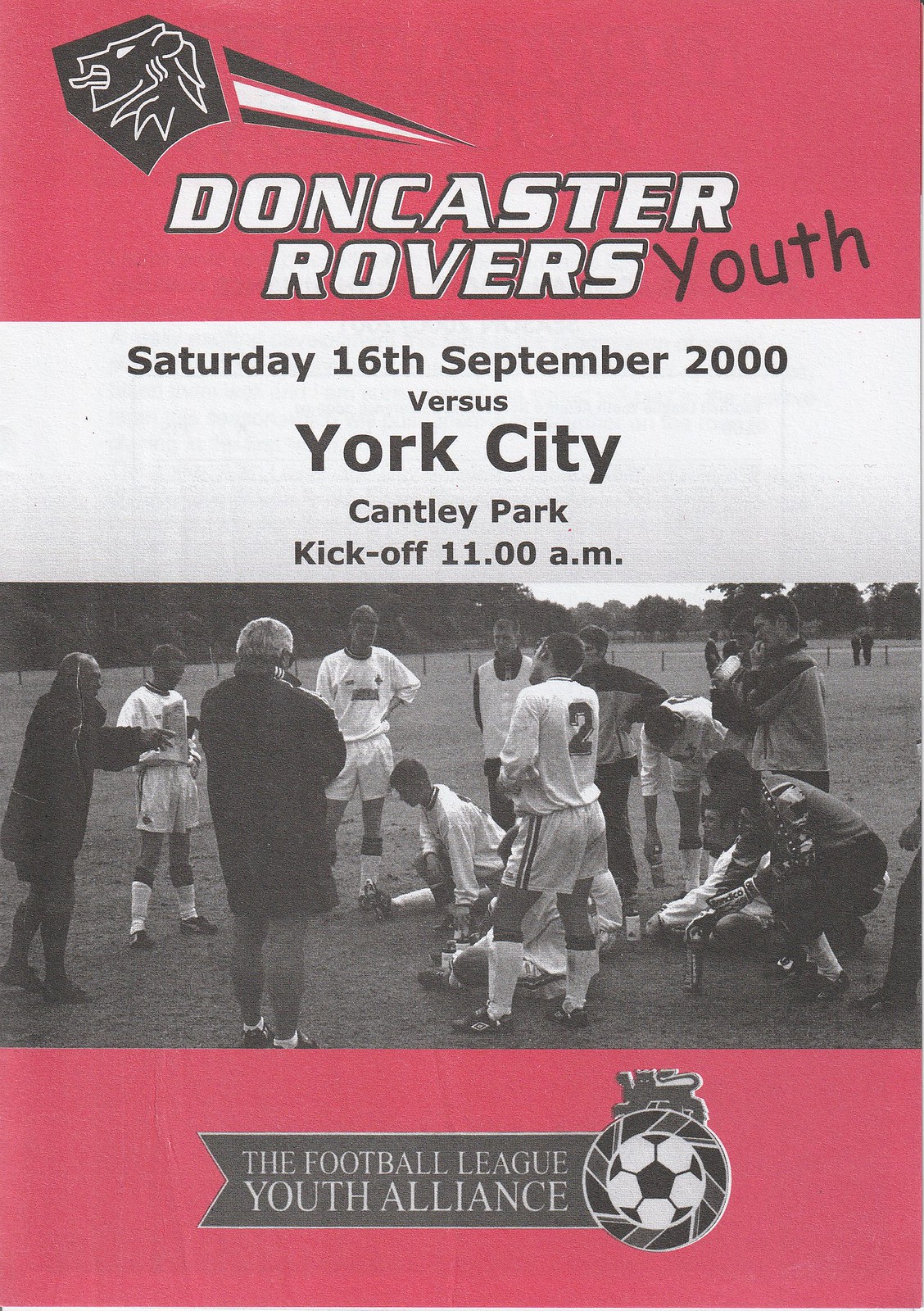The tall rectangular poster features prominent thick red rectangles at both the top and bottom. The top left corner showcases a white lion symbol etched onto a black background. Adjacent to it, in bold white block letters, are the words "Doncaster Rovers," followed by "Youth" in black font. Below this, within a white rectangle, details are presented in black font about the upcoming match: "Saturday, 16th September 2000 versus York City, Cantley Park, kickoff 11 a.m." The central part of the poster is dominated by a black and white photograph depicting a soccer team, clad in white jerseys and shorts, possibly engaged in a pre-game strategy discussion or post-game cool down. Coaches dressed in black can also be seen interacting with the players who are huddled together on a field. At the very bottom, on a ribbon, the poster notes "The Football League Youth Alliance" along with an emblem featuring a football and a lion. This detailed presentation informs viewers about the event while capturing the team’s camaraderie and preparations.